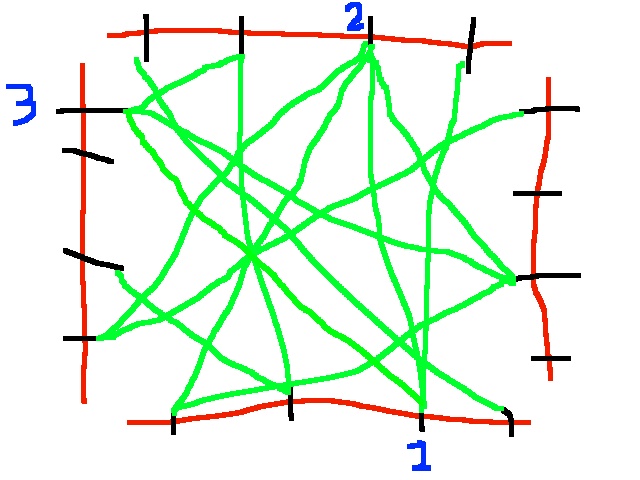The image depicts a geometric drawing on a white background comprised of interconnected red, black, blue, and green lines. There are four primary red lines: the bottom line, which arches slightly, the top line, which is mostly straight, a vertical line on the far left, and a slightly curved vertical line on the far right.

1. **Bottom Red Line**: 
   - Curved upwards slightly.
   - Intersected by four vertical black lines.
   - The third vertical black line from the left is marked with a blue number "1".

2. **Top Red Line**: 
   - Straight overall.
   - Also intersected by four vertical black lines.
   - The third vertical black line from the left bears a blue number "2".

3. **Left Red Vertical Line**: 
   - Perfectly straight.
   - Intersected by four horizontal black lines.
   - The topmost black horizontal line features a blue number "3".

4. **Right Red Vertical Line**: 
   - Slightly curved.
   - Intersected by four horizontal black lines.
   - No numbers are present on this line.

Inside the boundary formed by the ends of the black lines on the red lines, a complex mesh of green lines crisscrosses, connecting various points with seemingly no apparent pattern, creating a web-like structure within the red line framework.